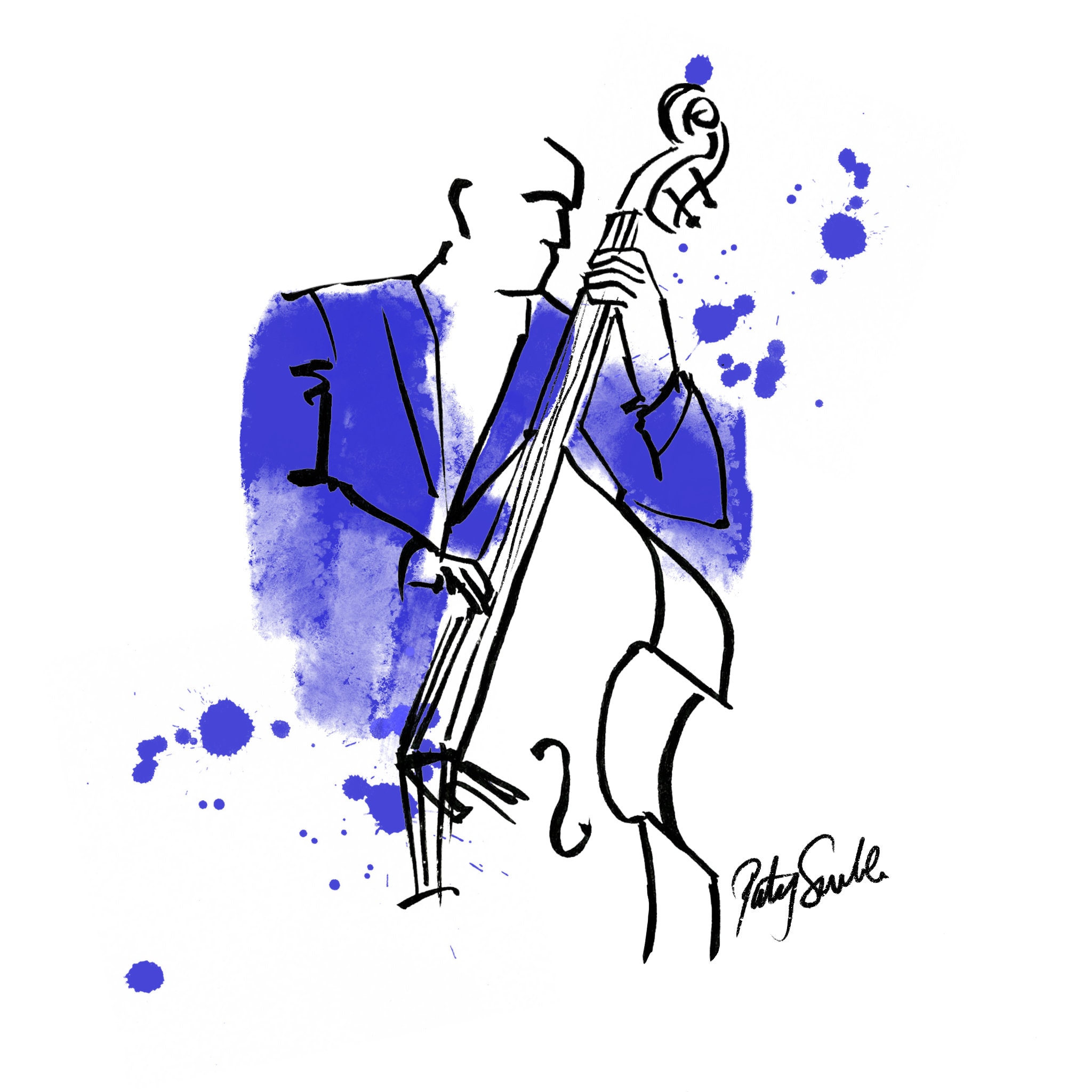The artwork features a man playing a cello, facing to the right with the cello positioned beside him. He's dressed in a vibrant blue suit that contrasts starkly against the monochrome black lines that comprise the rest of the piece. Splashes of blue paint add dynamic texture to areas of the artwork, enhancing the visual impact of his attire. The man's facial and physical details are hinted at rather than fully defined, lending a somewhat abstract quality to his depiction. The background is a crisp, solid white, bringing the central figures into sharp relief. Notably, the lower right section of the cello displays the artist's signature, although it's somewhat difficult to discern. This signature, along with the exaggerated height of the cello relative to the man, adds unique elements to the composition.